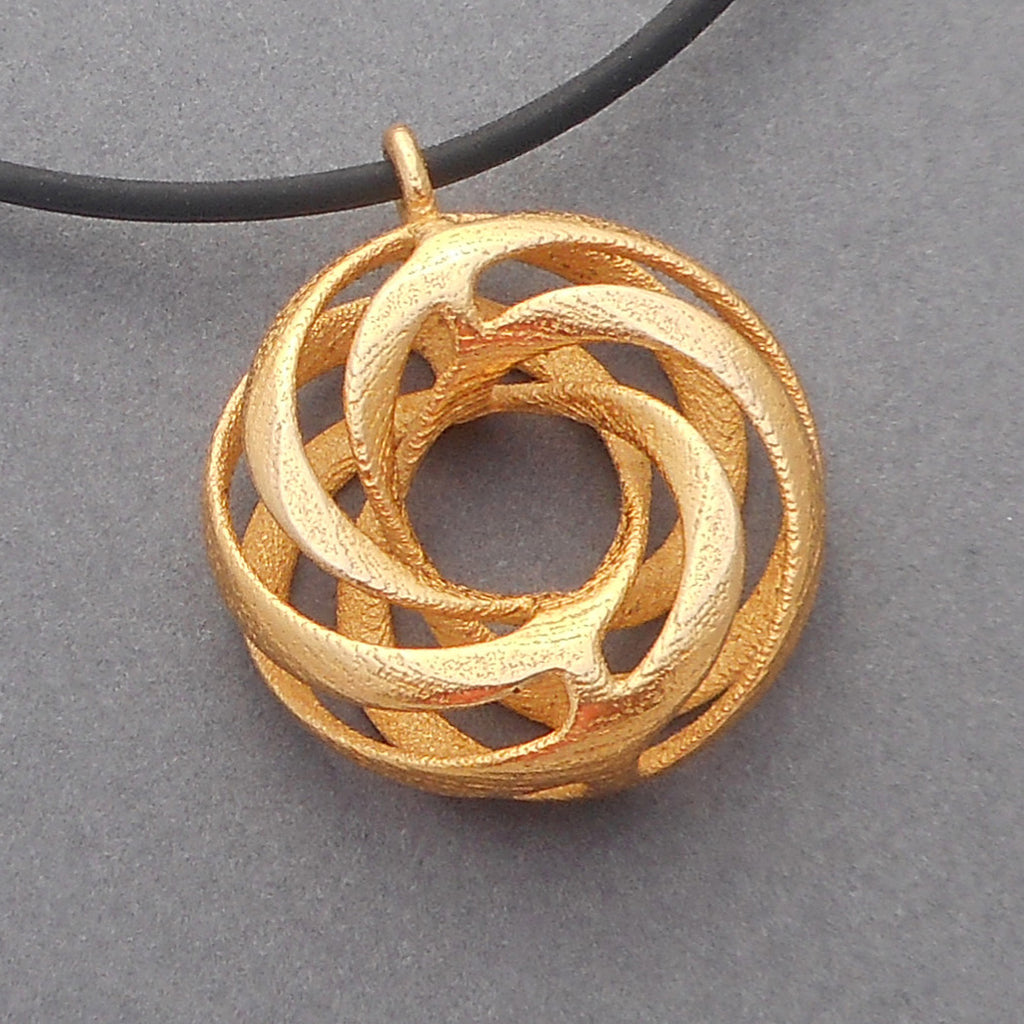The image showcases a close-up view of a gold jewelry pendant, prominently featured against a gray, possibly felt-textured background. The pendant, which is securely fastened to a somewhat thick black rope resembling a hair ponytail elastic, is three-dimensional and intricately designed. It consists of multiple layers of swirling circular patterns that converge at a small, empty central hole. These swirls are about four layers deep, creating a rich, ornate appearance. At the top of the pendant, a gold loop connects it to the black rope, highlighting the craftsmanship of the piece.